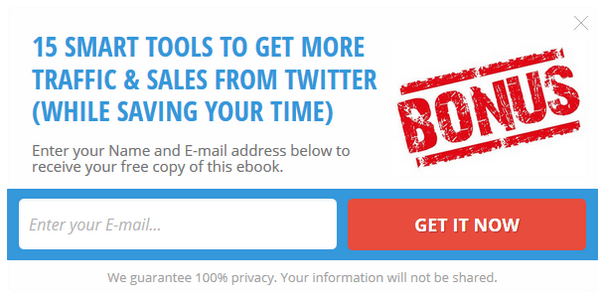Here is a cleaned-up and detailed caption for the given image:

The advertisement prominently features a bold blue heading in uppercase letters that reads "15 Smart Tools to Get More Traffic and Sales from Twitter (While Saving Your Time)." To the right of this, there is a red stamp-like graphic labeled "BONUS" in all caps. Below the heading, there is a prompt instructing readers to "Enter your name and email address below to receive your free copy of this ebook." 

A white email input field is highlighted by a blue rectangular box, where users can type in their email address. To the right of this field, a red button with the text "GET IT NOW" in uppercase letters invites users to submit their information. Beneath the submission area, a privacy assurance message states, "We guarantee 100% privacy. Your information will not be shared."

This web ad effectively promotes a free ebook offering "15 Smart Tools" to increase Twitter traffic and sales while requiring personal information, such as an email address, for access. Despite being advertised as free, the promotion suggests there may be additional costs involved in the future for similar offerings.